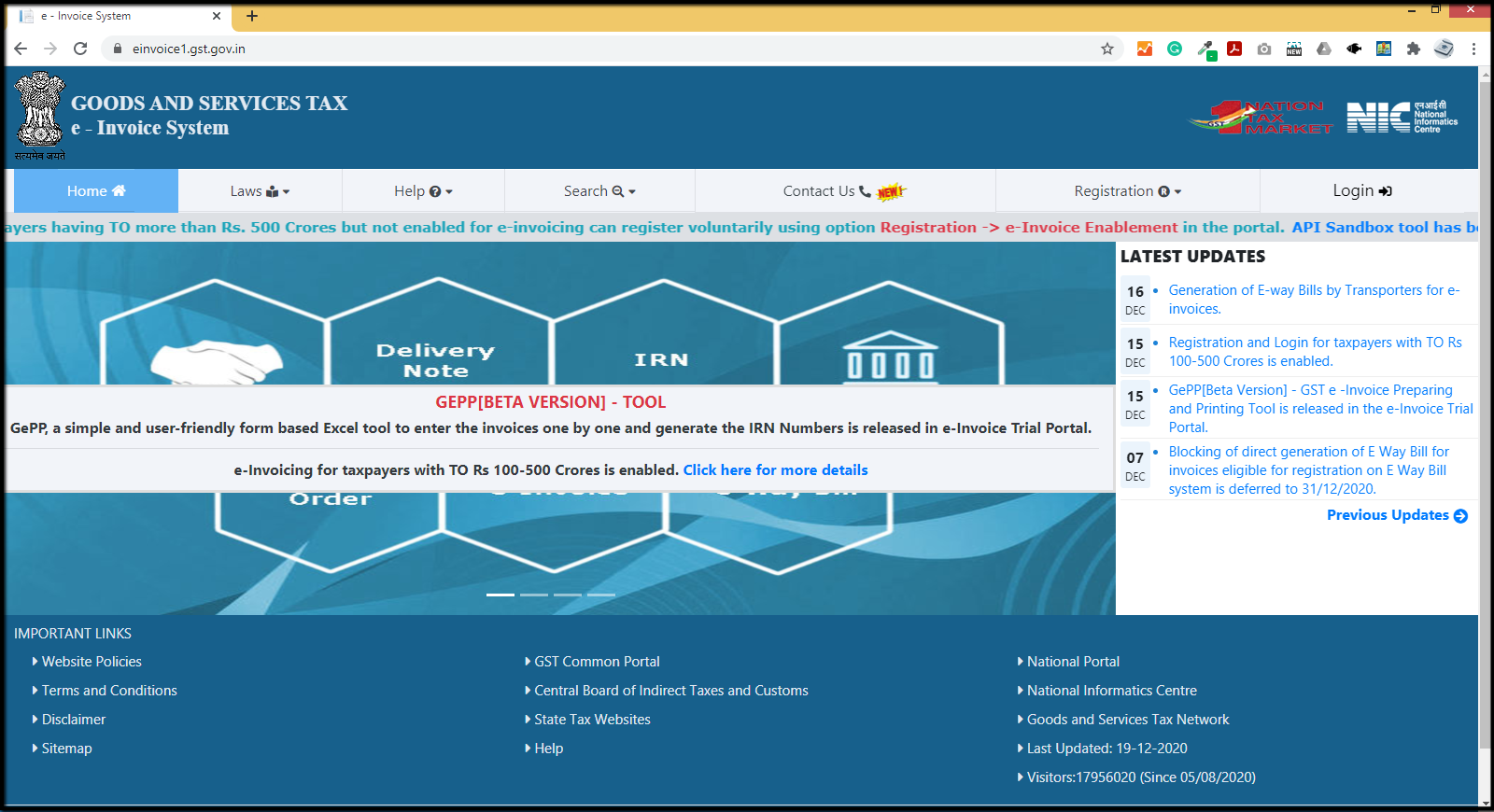The screenshot features a webpage that mimics the appearance of an official government site, specifically relating to the Goods and Services Tax (GST) eInvoice System. The webpage is titled "Invoice System" in the browser's tab, suggesting a focus on managing invoices electronically. The site prominently displays "Goods and Services Tax eInvoice System," "Nation Tax Market," "NIC," and "National Informatic Center," to reinforce its governmental theme.

The website's navigation bar includes tabs labeled Home, Laws, Help, Search, Contact Us, Registration, and Login, offering a structured layout for users. On the right-hand side, a section titled "Latest Updates" is displayed, highlighting the latest information such as the December 16th update regarding the generation of eWay bills by transporters for invoices, along with other unspecified dates.

Across the screen, there is a notice for the "GEP Beta Version Tool," described as a simple and user-friendly Excel-based form for entering invoices individually. However, caution is advised when using or trusting this site, as it mimics a governmental website but may contain hidden elements in the search bar or other areas that could signify it is not an official and secure source.